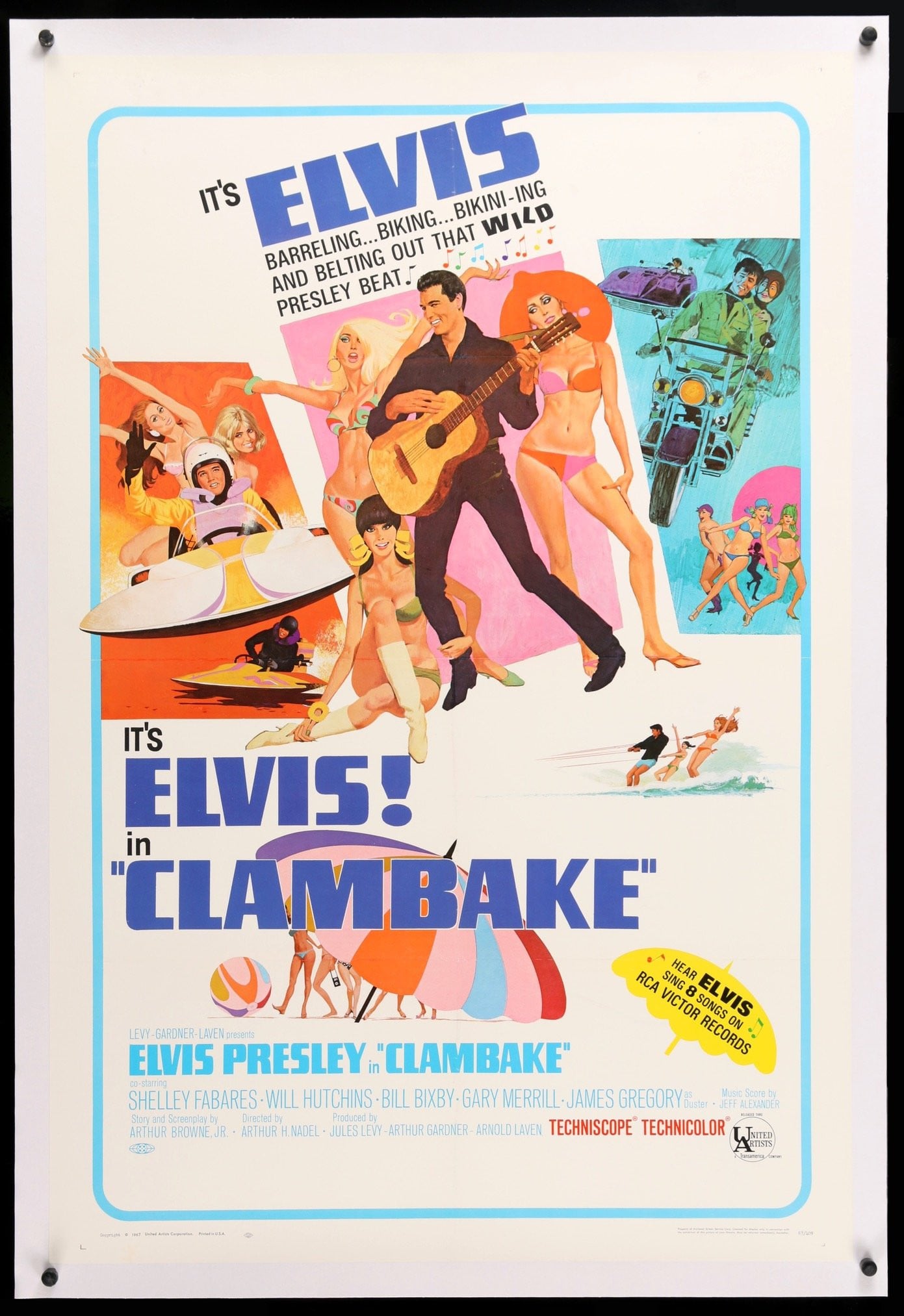The vertically oriented movie poster for "Clambake," featuring Elvis Presley, is prominently displayed in a black frame with a half-inch white border. The poster itself has a cream-colored background with an offset rectangular light blue line framing it. It showcases artist-rendered illustrations of Elvis in three distinct scenes. 

In the first scene, rendered against a blue background, Elvis is riding a motorcycle with a girl seated behind him. The middle scene, set against a pink background, depicts Elvis dressed entirely in black, playing a guitar with three girls in bikinis dancing around him. In the third scene, Elvis is seen driving a speedboat with two girls behind him, likely in the context of a Clambake party.

The poster prominently features the text: "It's Elvis, barreling, biking, bikini-ing and belting out that wild Presley beat," followed by "Elvis in Clambake" beneath it. At the very bottom, within a small yellow umbrella graphic, it promotes Elvis's eight songs available on RCA Victor Records. Further credits include co-stars Shelly Fabre, Will Hutchins, Bill Bixby, Gary Merrill, and James Gregory, and it highlights the movie's Technicolor and Techniscope formats. Several scenes also show multiple bikini-clad women in various playful and celebratory poses, enhancing the fun and lively atmosphere of the film.